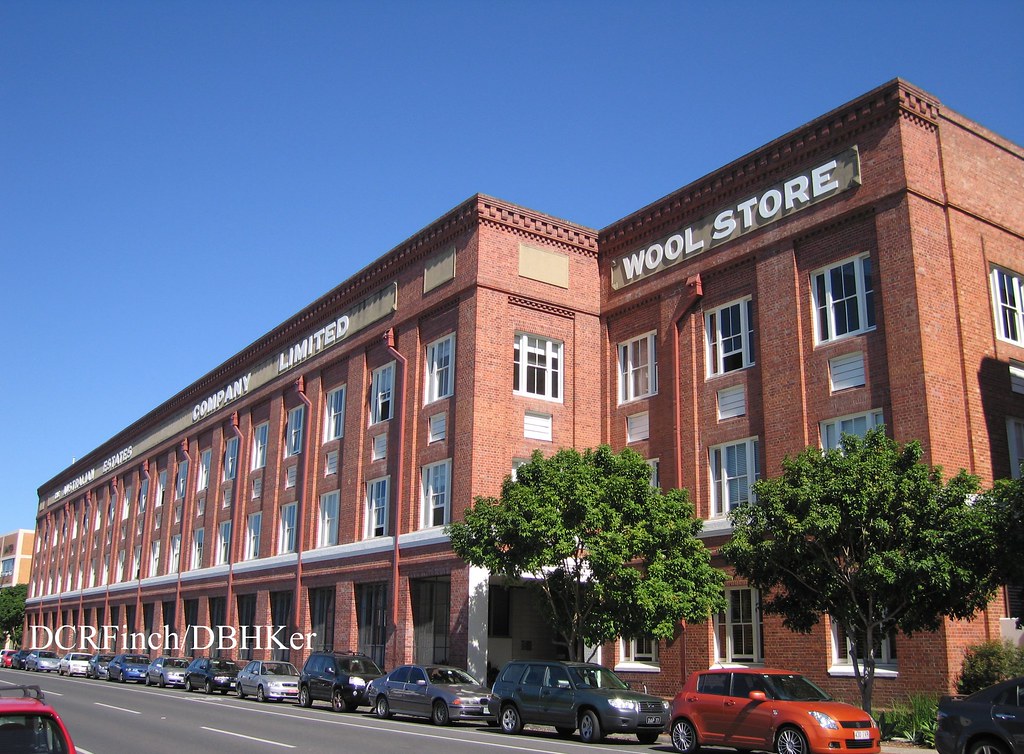This color photograph, credited to D.C.R. Finch and D.B.H. Kerr from their watermark, captures a large red brick building identified as the Metropolitan Estates Company Limited Wool Store. The building's facade features a very continuous and regular pattern, stretching across its three stories. The first floor has one window, the second floor has a window with blinds, and the third floor includes another window flanked by a small white vent. Prominent white text spelling "Metropolitan Estates Company Limited" spans the front, with "Wool Store" marked prominently on the top right corner.

In front, a street lined with a variety of parked cars runs parallel to the building; there are approximately 13 to 15 cars facing to the right. The scene illustrates urban greenery with two sizable trees directly in front of the store and additional trees in the background, suggesting a tree-lined street. This meticulously captured image emphasizes both the architecture of the building and its bustling urban environment.